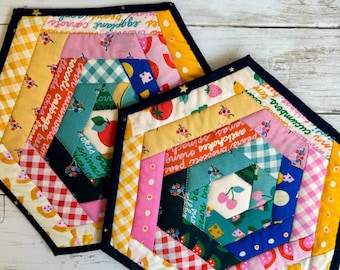The image showcases two hexagonal quilted pot holders, each with intricate, colorful designs and a black border. Both pot holders feature a combination of checkered yellow and white, checkered red and white, and green sections. The pot holder on the left has a central apple motif, while the right one displays a pair of cherries. Surrounding these central fruits are various patterns, including depictions of fruits and vegetables labeled with their names, such as artichokes, peas, broccoli, cucumbers, and eggplants. The pot holders are positioned on a silver and white striped table, set against a gray hardwood floor, with the right pot holder tilted at a 30-degree angle counterclockwise.